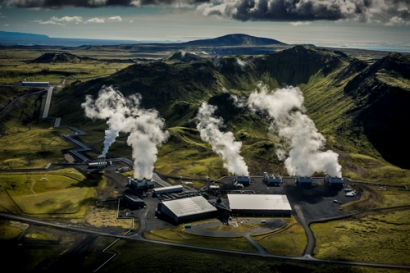This aerial photograph captures a small, sprawling industrial facility, likely a power plant or factory, nestled within a lush green valley. The facility comprises several warehouses and at least four large buildings, prominently featuring smokestacks venting significant amounts of exhaust or steam. The scene is framed by a semicircular mountain range immediately behind the buildings, with additional mountains and tall hills visible further in the distance. The area is crisscrossed by various roads, emphasizing its industrial activity. The sky above presents a mix of white puffy clouds and darker, more ominous grayish clouds, though natural light still illuminates the ground below. Despite the photo's small size and high vantage point making finer details hard to discern, the overall composition clearly highlights an expansive industrial complex set against a picturesque, mountainous backdrop.